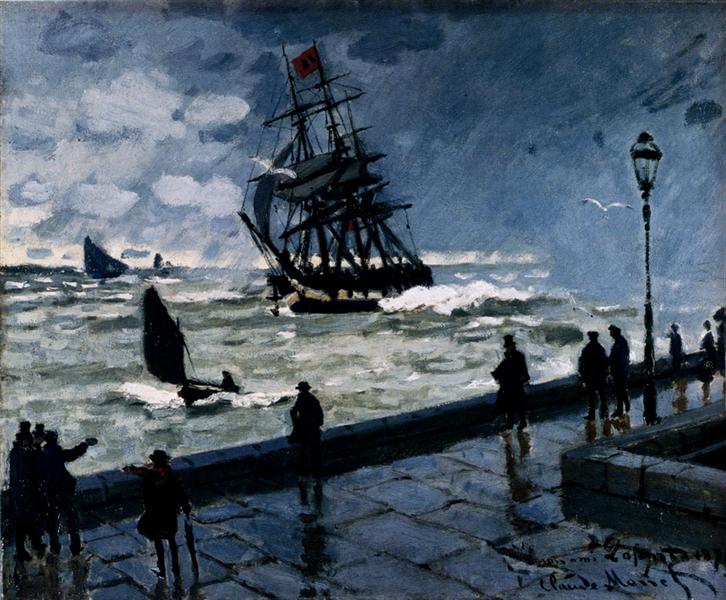This impressionistic oil painting vividly captures a nocturnal maritime scene with a large old-fashioned sailboat navigating choppy, rough waters. The boat, equipped with rigging and a few sails, is surrounded by several smaller boats amidst waves cresting with whitecaps. The dark, stormy sky overhead is filled with an array of blue, gray, and almost black clouds that suggest impending rain, particularly on the right side of the horizon where intermittent brushstrokes depict rainfall. Adjacent to the turbulent sea is a dark cobblestone pathway featuring the silhouettes of several dark-clad figures, some of whom appear to be wearing hats, including one resembling a top hat. These figures stand gazing out over the waterfront, illuminated by an old-fashioned light pole that casts a subtle glow over the scene. A signature at the bottom right corner of the painting bears the name Claude Manet, subtly anchoring the piece's authenticity.